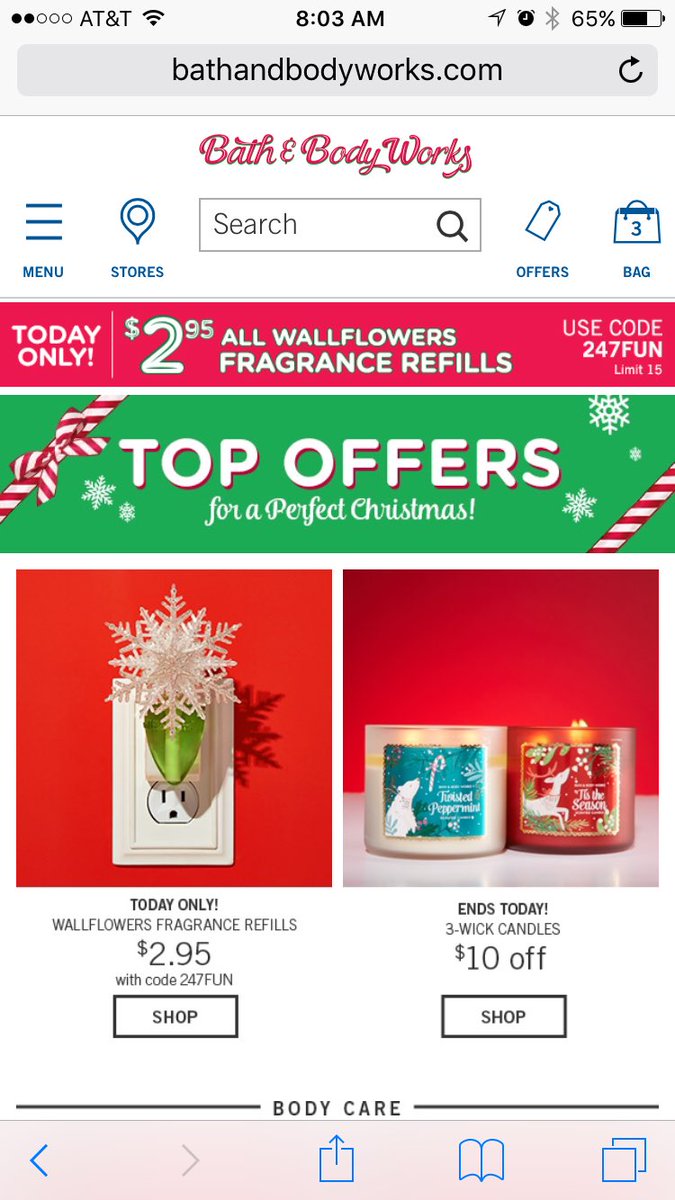A vertical image captured from a smartphone screen displays a webpage, specifically an advertisement from Bath & Body Works. The top portion of the screen reveals the smartphone's status bar showing a light gray strip, with two filled circles on the upper left, indicating some in-progress activities. The status bar also mentions the carrier, AT&T, accompanied by a Wi-Fi symbol. Centrally, the time is displayed as 8:03 a.m., and on the upper right, various icons are visible, including Bluetooth, a clock, and a battery life indicator at 65%.

The URL bar right below the status bar reads "bathandbodyworks.com," alongside a reverse arrow icon indicating a back function. Below this, the webpage header includes the Bath & Body Works logo in red, a menu button, a stores link, a search bar with a magnifying glass icon, an offers tab, and a shopping bag icon showing three items.

Prominently featured on the webpage is a promotional banner stating: "Today Only: $2.95 on All Wallflowers Fragrance Refills, Use Code 247FUN, Limit 15." The banner is decorated with festive elements like green boxes, snowflakes, and red-and-white candy cane stripes. Below this promotion, another highlighted offer reads: "Top Offers for a Perfect Christmas - Today Only, Wallflowers Fragrance Refills $2.95 with Code 247FUN," followed by a "Shop" button. Another promotion indicates, "Ends Today: Three Wick Candles $10 Off," accompanied by another "Shop" button.

In the middle section, separated by two black horizontal lines, a "Body Care" label is displayed in black text. The bottom of the webpage features typical browser navigation icons including a share button, bookmarks, and forward and backward arrows.

This detailed image captures the holiday promotional offers available on Bath & Body Works' mobile website, tempting shoppers with limited-time deals on fragrances and candles.